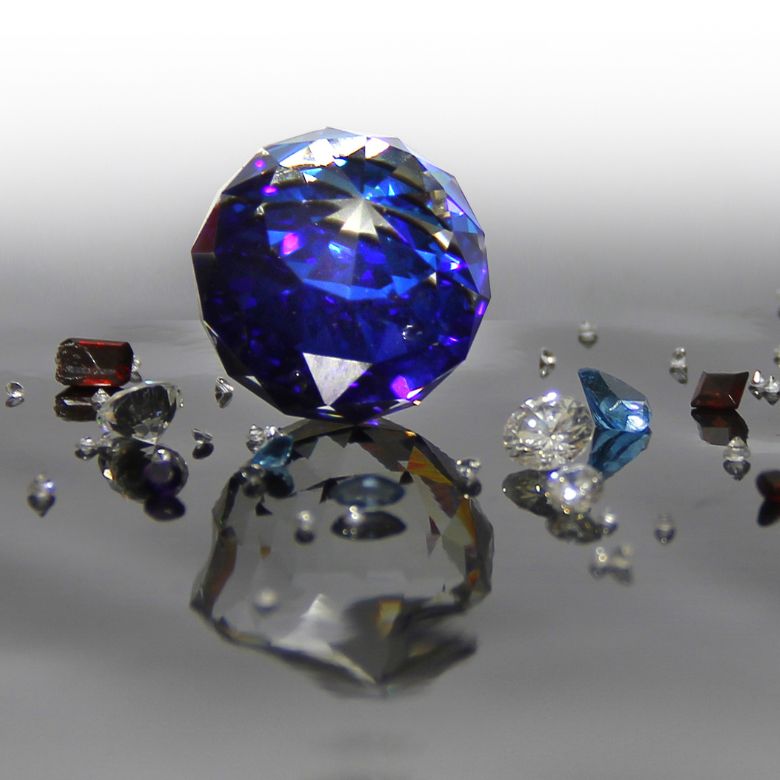This square image showcases an array of gemstones displayed on what appears to be a reflective glass surface. The background transitions from a near-white at the top to a darker gray at the bottom, enhancing the clarity and brilliance of the jewels. Dominating the center is a large, round, blue gemstone that strongly resembles a sapphire, notable for its vibrant blue hue with intriguing reflections of silver and black, and hints of purple. Surrounding the central sapphire are several smaller gemstones: on the right, there is a collection of tiny clear diamonds and a lighter blue jewel, potentially an aquamarine. To the left of the sapphire, there is a square-cut red ruby accompanied by additional small diamonds. The reflections of these gemstones are clearly visible on the glass surface, adding to the visual complexity and elegance of the photograph.